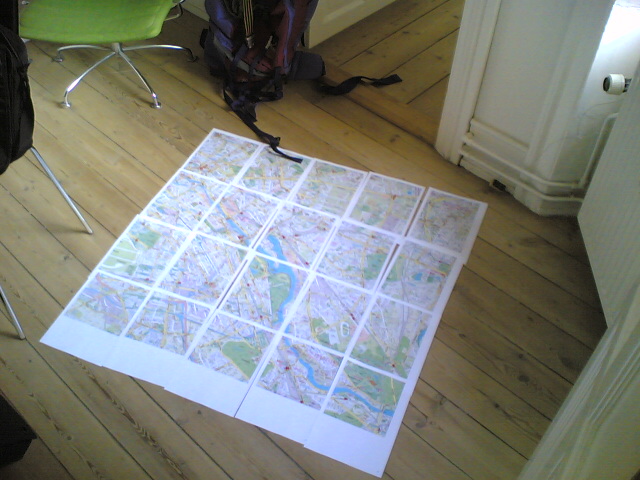The image is a detailed, high-angle color photograph of a large composite map, meticulously laid out on a wooden floor in a 5 by 4 grid formation. Each section of the map is printed on individual A4 white paper sheets, pieced together to create a larger, cohesive whole that depicts roads and rivers seamlessly transitioning across the grid. The scene is likely set in a room with a white-painted wooden finish on the walls, possibly a dining room.

In the top left corner, a lime green office chair with thin, rounded metal legs is prominently visible. Adjacent to it, on the left edge, there is a hint of a black chair, also supported by thin metal legs. In the middle top of the image, a black and purple backpack or rucksack with visible straps is leaning against the doorway, which opens out into another room or hallway. This doorway, with a white door slightly ajar, reveals more wooden flooring and possibly a window beyond, allowing light to filter through.

To the right side of the picture, the wooden floor transitions into a cream-colored area, which may contain furnishings like a radiator, indicated by a small round object and some wall paneling at the bottom. The careful arrangement of the map sheets on the floor, alongside the visible preparations and items like the backpack, suggest that someone is planning a trip or a holiday.